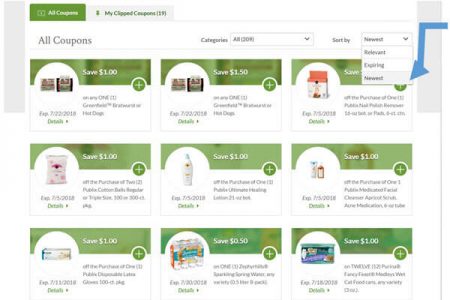This image depicts a coupon website with a predominantly green and white color scheme. In the upper left corner, there are two tabs: the first tab is green with the text "All Coupons" written in white, while the second tab is white with the text "My Clipped Coupons" and a number in parentheses, likely indicating the count of clipped coupons, which appears to be 19. To the right of these tabs, near the top of the page, there is a drop-down box with sorting options that include "Newest," "Relevant," and "Expiring," among other options that are partially obscured. A blue arrow is pointing at the last entry in this drop-down.

Below the two tabs in the top left section, under the "All Coupons" label, there is another drop-down box centrally aligned. The display area features three rows, each containing three coupons. The top half of each coupon is green, while the bottom half is white. On the right side of each coupon, there is a plus symbol for adding or clipping the coupon. Above this symbol, the amount of money saved with each coupon is displayed in white text.